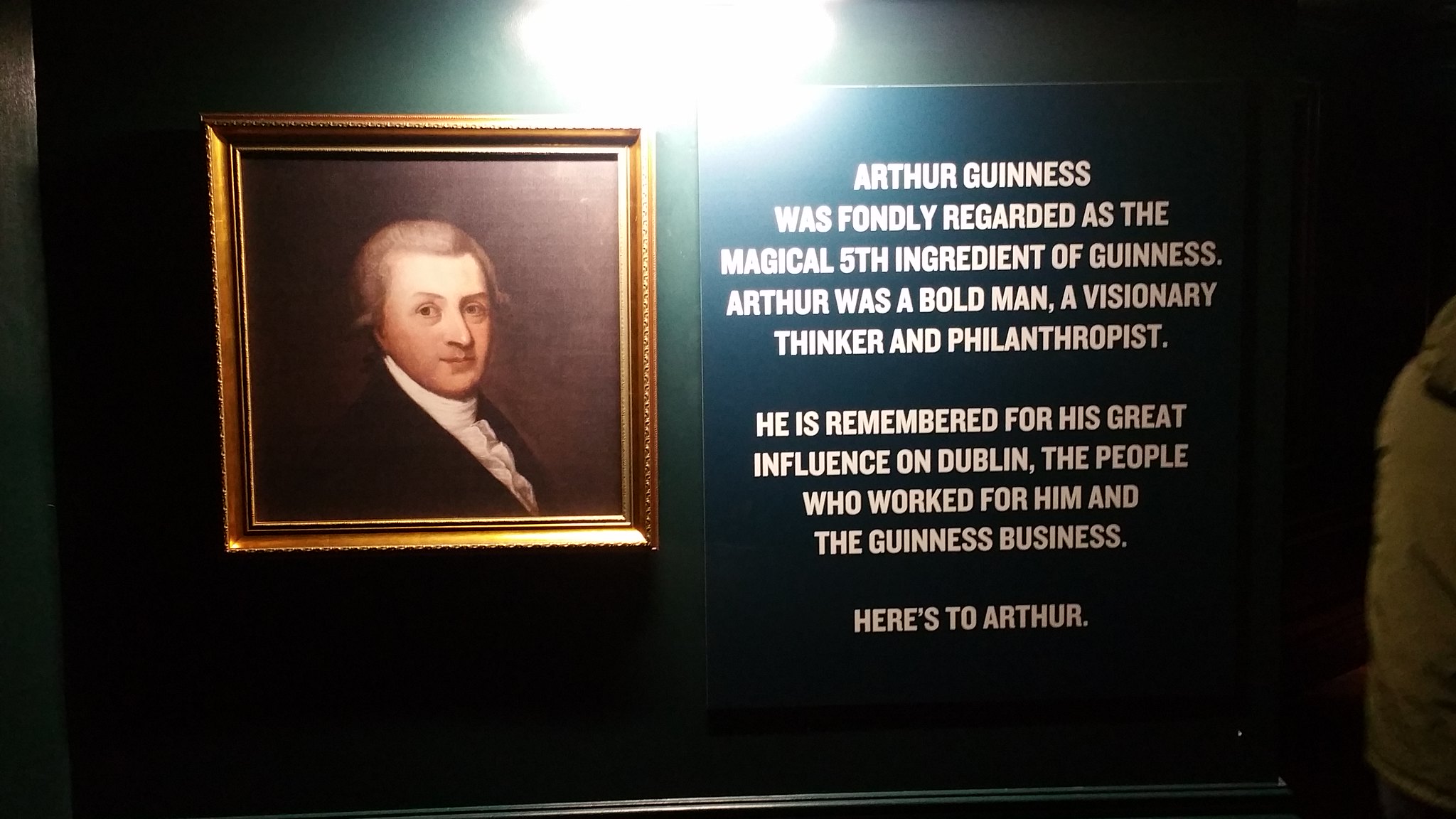This photograph captures a richly detailed portrait within an ornate gold frame, set against a dark background that appears black or deep blue. Illuminated by overhead light, the painting emits a soft glow. The subject, Arthur Guinness, depicted in period attire with a frilled white shirt and dark jacket, gazes slightly over his right shoulder. To the right of the portrait, white text honors Arthur Guinness, describing him as the "magical fifth ingredient of Guinness." The inscription celebrates him as a bold man, visionary thinker, and philanthropist, praising his significant influence on Dublin, his employees, and the Guinness business. The heartfelt tribute concludes with "Here's to Arthur."